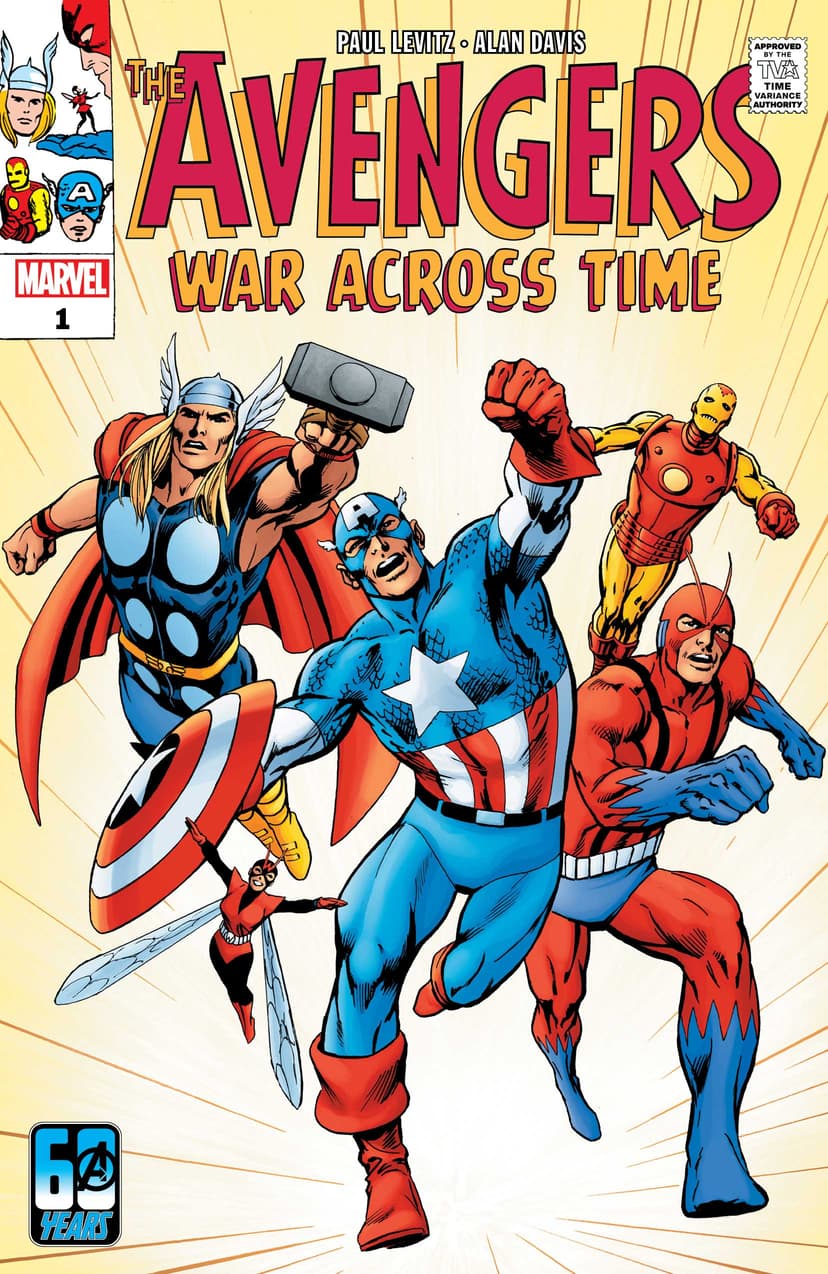This vibrant comic book cover belongs to the Avengers series and features dynamic action figures against a striking backdrop. At the top, in bold red letters with yellow highlights, is the title "The Avengers," with the subtitle "War Across Time" just below it in matching colors. The authors, Paul Levitz and Alan Davis, are credited at the top in white text.

Dominating the center of the cover are four iconic characters. Captain America stands prominently, his blue uniform adorned with a white star, and his white-gloved hand forms a determined fist. To his left is Thor, recognizable by his winged helmet and gray hammer clenched in his fist. To the right is Ant-Man, dressed in an ant-like costume with blue gloves and boots, while Iron Man stands vigilant in his own distinctive suit. Additionally, Wasp is depicted in the lower left corner, contributing to the ensemble of heroes.

On the top left portion, a white lens displays the Marvel logo above a black number one, indicating this is the first issue. The cover is framed by a red background with the faces of some characters adding to the action-packed visual. The logo "60 years" in blue and black is positioned towards the bottom left, celebrating the comic's long legacy.